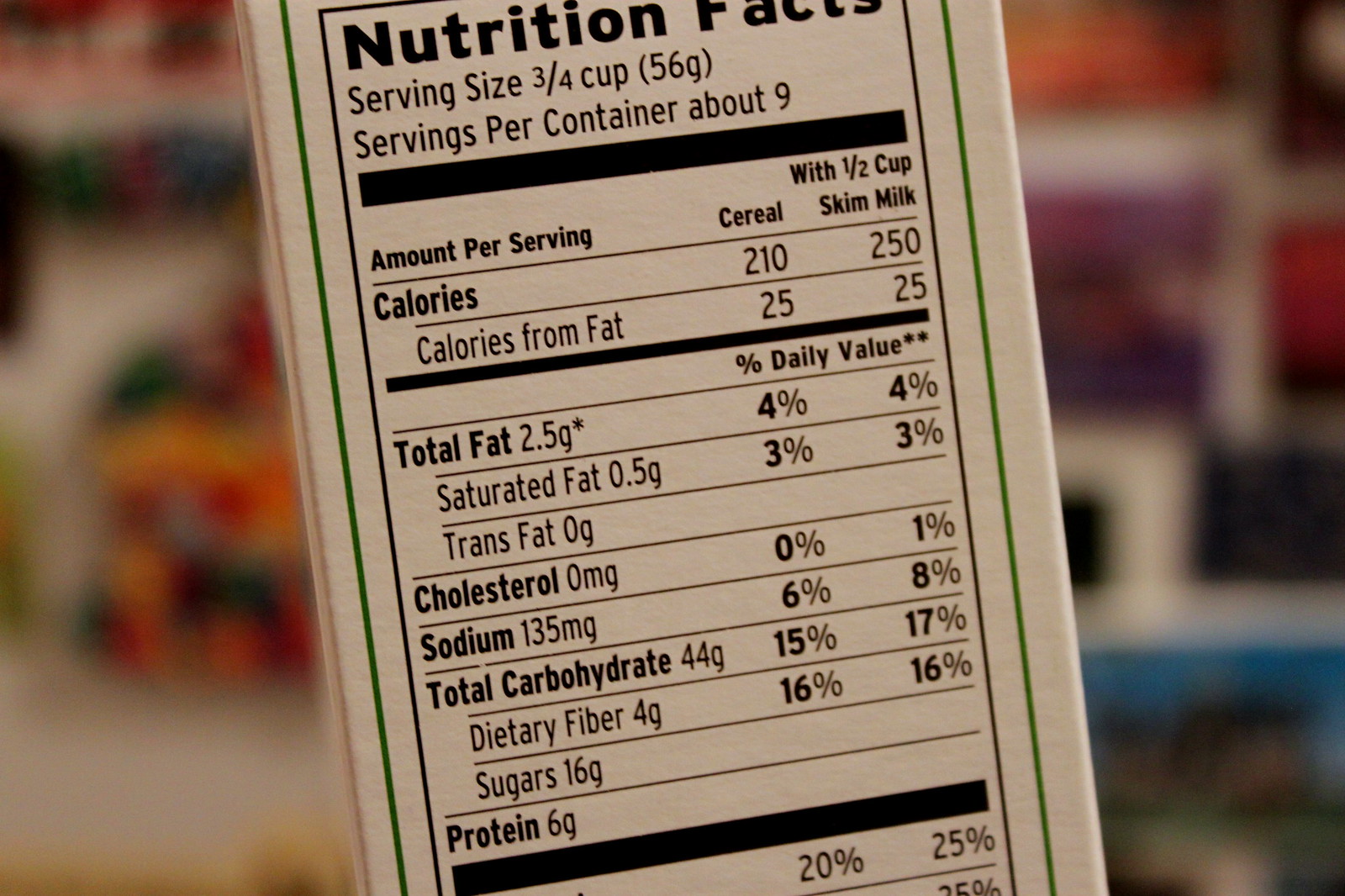This horizontal image provides a detailed close-up of the nutrition facts label on a white box. The information is printed in clear, black lettering and is organized in a tabular format. The label indicates that the serving size is three-quarters of a cup, with approximately 9 servings per container. It specifies that the cereal alone contains 210 calories, which increases to 250 calories when consumed with half a cup of skim milk. The total fat content is listed at 4% of the daily value, with cholesterol at 0%. Sodium levels are marked at 6%, total carbohydrates at 15%, and dietary fiber at 16% of the daily value. Additionally, the label notes that there are 16 grams of sugar and 6 grams of protein per serving.